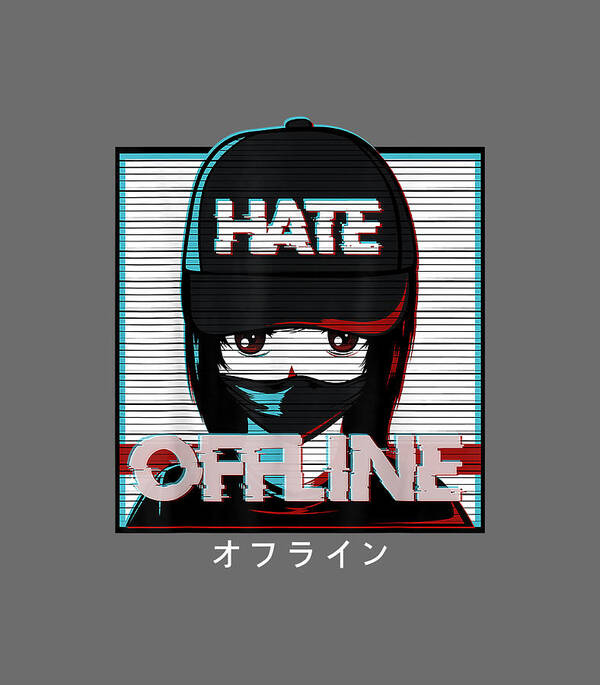The image is a detailed piece of anime-style artwork framed by a medium gray border with a black and light blue outline. At the center is a pale-skinned character with long hair, highlighted in red on the right and blue on the left. The character wears a black baseball cap featuring the word "HATE" in bold white capital letters, with blue and red accents. The character's expressive brown eyes peek out from above a black face mask. The background showcases black and white horizontal lines, adding a glitch effect by incorporating blue and red areas. Beneath the character's face, the word "OFFLINE" appears in large uppercase light pink letters. The character is dressed in a black outfit with hints of red and blue, and below the word "OFFLINE," there are white Asian characters completing the composition.